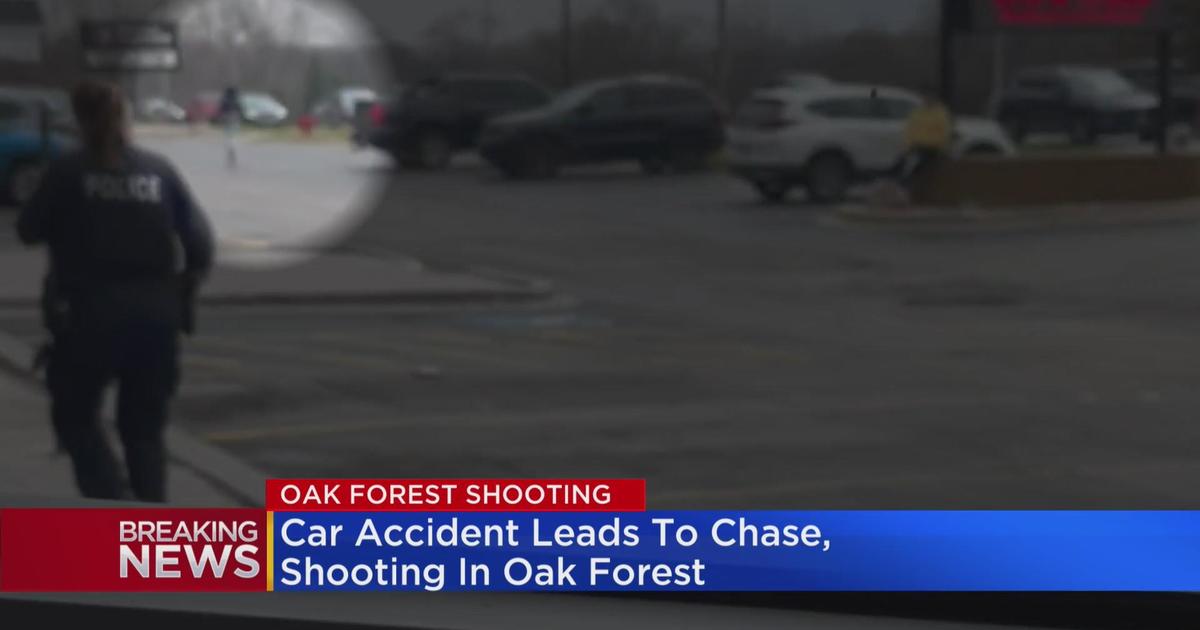This image is a dark, grainy still from a televised news broadcast covering a breaking news story titled "Oak Forest Shooting." The text at the bottom of the screen, displayed in white letters on a red and blue banner, reads: "Breaking News. Oak Forest Shooting. Car accident leads to chase, shooting in Oak Forest." In the scene, there is a parking lot with multiple cars visible—three directly in front and several more parked perpendicular in the background. The image features a police officer on the far left, identifiable by the word "POLICE" written on the back of their dark blue uniform and a holster at their right hip. This officer appears to be walking away from the camera. Towards the right side of the image, there's a white vehicle, and near it, a person wearing a yellow jacket is standing or sitting. The focal point of the still is a lighter, white-circled area highlighting a blurred figure running away, presumably the suspect involved in the shooting incident. The entire scene is intentionally dim, directing attention to the circled area.